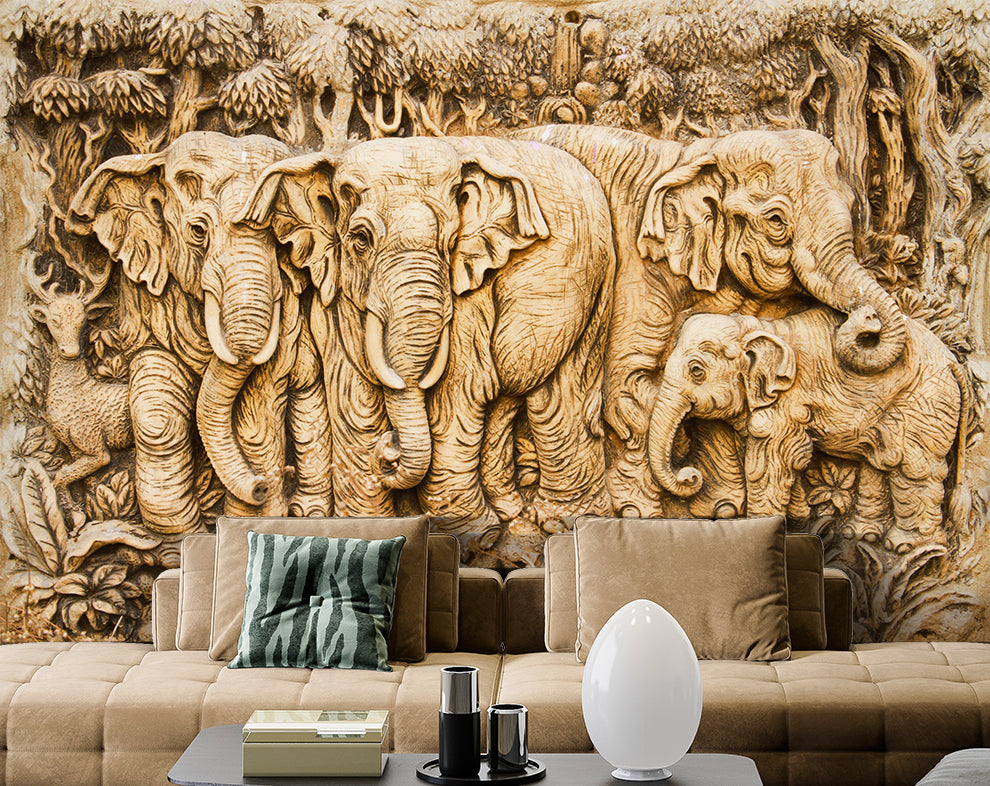In the photo of the lounge room, there's a striking wood-carved artwork mounted on the back wall. The intricate carving depicts a realistic scene with three large elephants and one baby elephant. Two of the elephants, which have visible tusks, are facing forward, while another large elephant looks away, its trunk resting gently on the baby elephant. To the left of the scene, a deer with antlers gazes in the same direction as the elephants. Dense foliage and trees, along with various ferns and flowers, are also carved into the background, adding depth to the vista.

Below this detailed carving is a plush, coffee-colored velvet couch adorned with four brown velvet pillows and a contrasting black and gray zebra-pattern pillow on the left side. The couch spans the width of the scene and provides a cozy seating area.

In the foreground, a black coffee table holds a collection of items: a distinct white egg-shaped object that appears to be a light, a shaker cup combo, and a metal box. This detailed arrangement gives a glimpse into a stylishly decorated and comfortable living space.